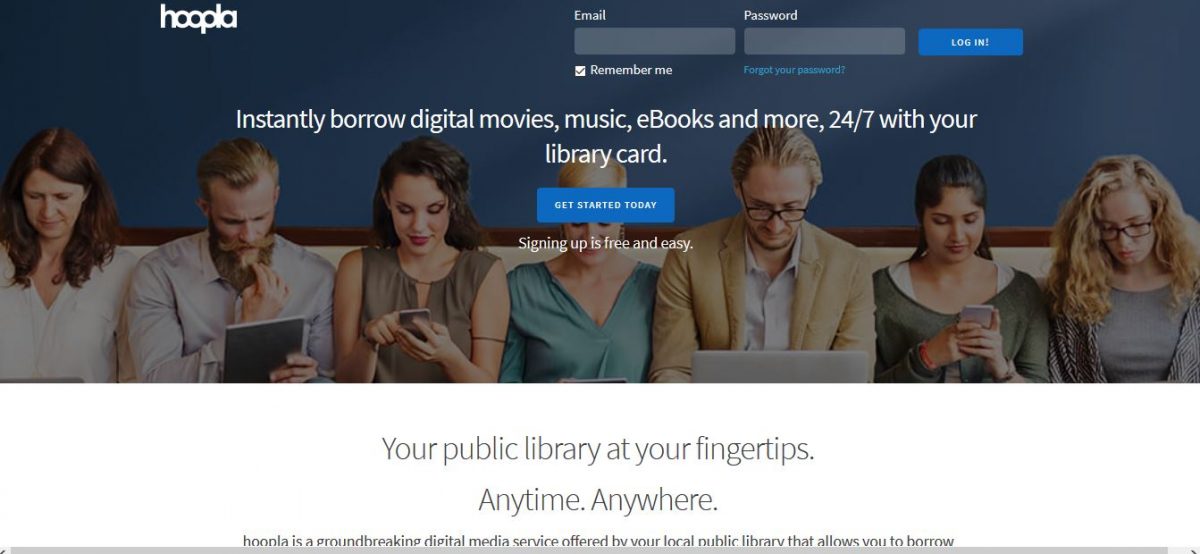This portrait-oriented image captures the homepage of a website called "Hoopla." The photo is long and narrow, with an approximate aspect ratio of 2 to 2.5 times its height. At the top left, "Hoopla" is prominently displayed in white against a deep blue background that resembles either a chalkboard or a window.

The top center and right sections feature login fields—an email box and a password box, each labeled with "Email" and "Password" in white font within a gray box beneath them. Below the email box, a white check box is labeled "Remember Me." Beneath the password box, there's a blue hyperlink that reads "Forgot Your Password." To the right of these input fields is a long, rectangular blue button with the white text "Log In."

Just below the login section, white text on the blue background reads: "Instantly borrow digital movies, music, ebooks, and more 24/7 with your library card." Another long, rectangular blue button with white font underneath that invites users to "Get Started Today," accompanied by the subtext: "Signing up is free and easy."

The background features an image of seven people seated in a row, alternating between women and men. They appear engrossed in various digital devices like phones, eBooks, and laptops. 

At the bottom of the image, gray text states: "Your public library at your fingertips, anytime, anywhere."